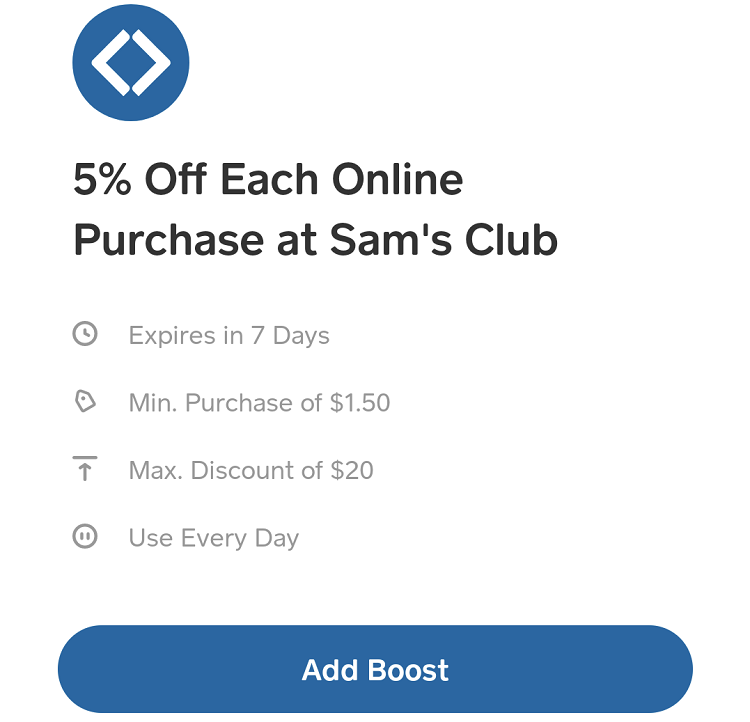The image showcases a coupon page for an app or website against a stark white background. At the top left corner, there is a blue circular icon featuring two nearly-touching arrows pointing in opposite directions, resembling a mathematical symbol, which creates a diamond-like negative space at their intersection. Below this icon, bold black text announces a "5% off each online purchase at Sam's Club." Directly underneath, a simplistic gray clock icon is accompanied by the expiration note, "expires in 7 days." A price tag icon follows, specifying a "minimum purchase of $1.50." Next in order is an arrow pointing upwards with a horizontal line above it, indicating a "max discount of $20." Below this, a circle icon with two small, vertical lines denotes that you can "use every day." Finally, at the bottom of the page, there's a prominent, pill-shaped button with a blue background matching the icon color, and white text that reads, "Add Boost."